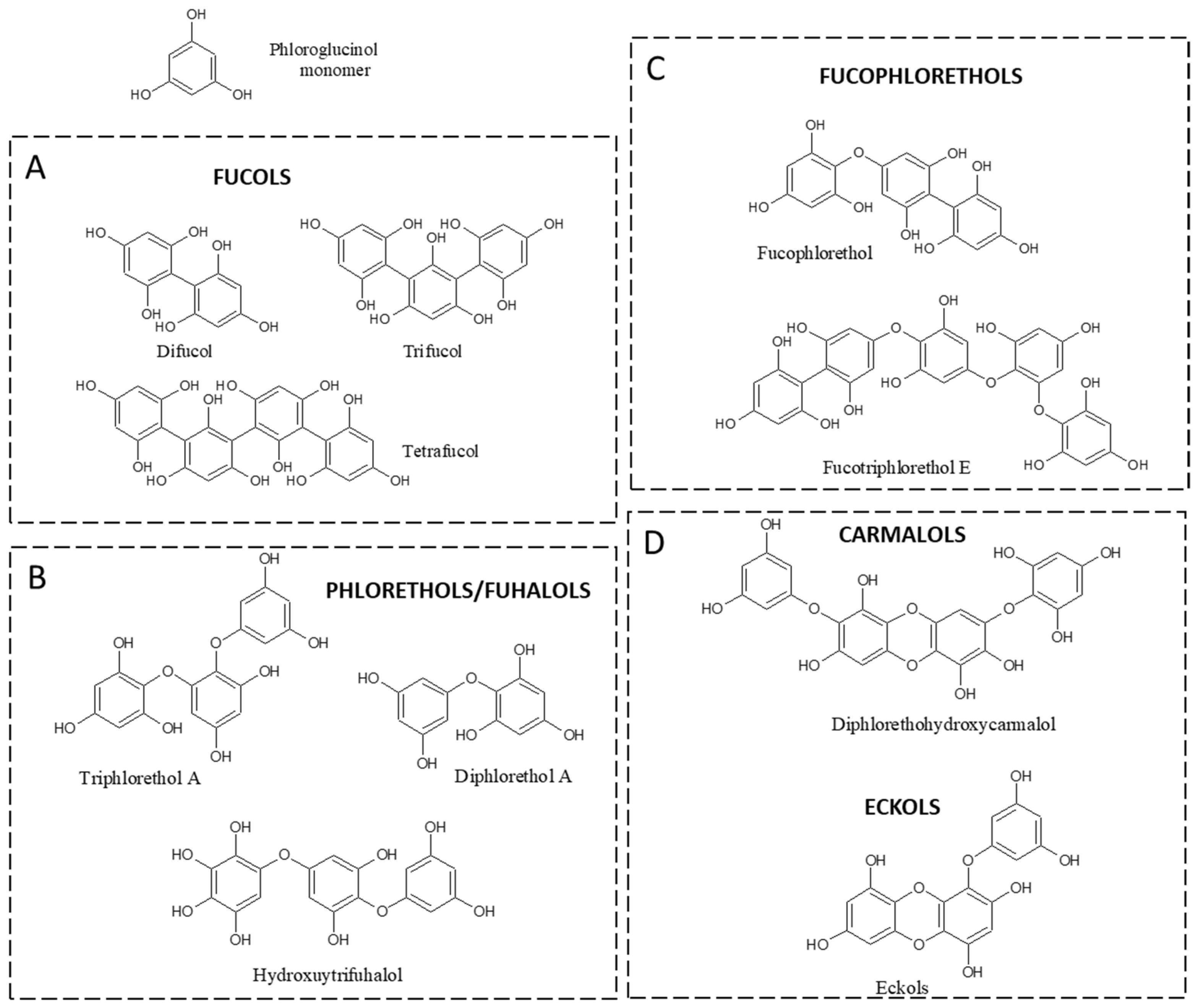The image presents four detailed diagrams, labeled A, B, C, and D, each depicting the molecular structure of various chemical compounds. Diagram A, titled "Fucols," illustrates three specific molecular structures comprising elements like oxygen, hydrogen, and possibly nitrogen, indicative of an organic compound. Diagram B is labeled "Fluorothals and Fuholals," while Diagram C is titled "Fucofluorothals." Lastly, Diagram D is labeled "Carmelols and Eckols," featuring another distinct set of organic compounds. Each diagram includes a series of lines and periodic table symbols to represent the chemical makeups of these compounds.